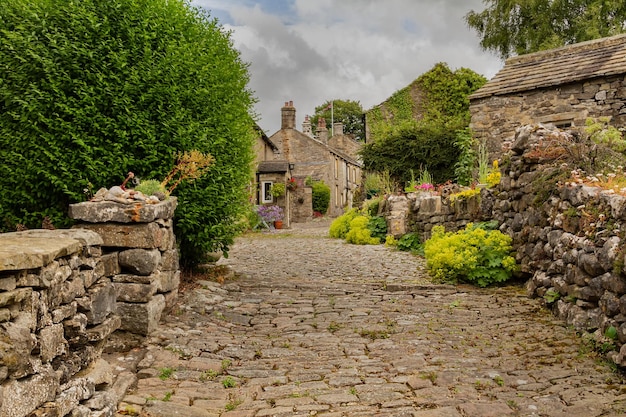This image showcases a quaint, old-fashioned village that evokes the charm of a European or British countryside. A worn cobblestone path leads the viewer's eye into the village, bordered by timeworn stone walls adorned with cascading plants and moss. Dominating the left side of the image is a giant, lush green bush, adding a vibrant touch to the scene. As we follow the path, a series of stone buildings come into focus. A prominent structure with multiple chimneys and floral decorations stands at the center, embodying the vintage aesthetic of the village. To its right, another stone building is enveloped in ivy and accompanied by a small tree in front, while a third stone building peeks from behind, partially obscured but revealing its weathered roof. The neat yet historic ambiance of the pathways, stone structures, and greenery, including patches of moss and ivy, creates a picturesque and serene setting reminiscent of classic European charm and tranquility.